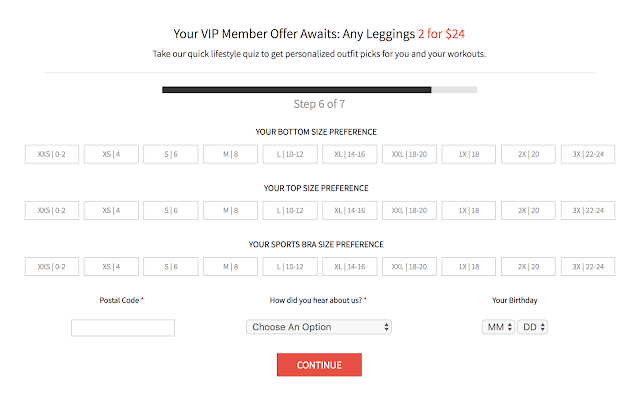A screenshot from a website detailing a special offer for VIP members is shown. The top of the image prominently features the text, “Your VIP Member Offer Awaits: Any Leggings Two for $24.” Below that, there's an invitation to "Take our quick lifestyle quiz to get personalized outfit picks for you and your workouts."

The image further indicates that the user is on "Step 6 of 7," which focuses on preferences for various clothing sizes. It begins with "Your bottom size preference," listing options from "Extra Extra Small (XXS)" up to "3X." This is followed by "Your top size preference," also offering sizes from "Extra Extra Small (XXS)" to "3X." Similarly, it includes "Your sports bra size preference" with the same size range.

Beneath the size preferences, there are fields for input, including "Postal Code" and a drop-down menu labeled "How did you hear about us? Choose an option." The final entry field on this step is "Your Birthday."

The layout is clean and organized, visually guiding users through the form to ensure a customized shopping experience.